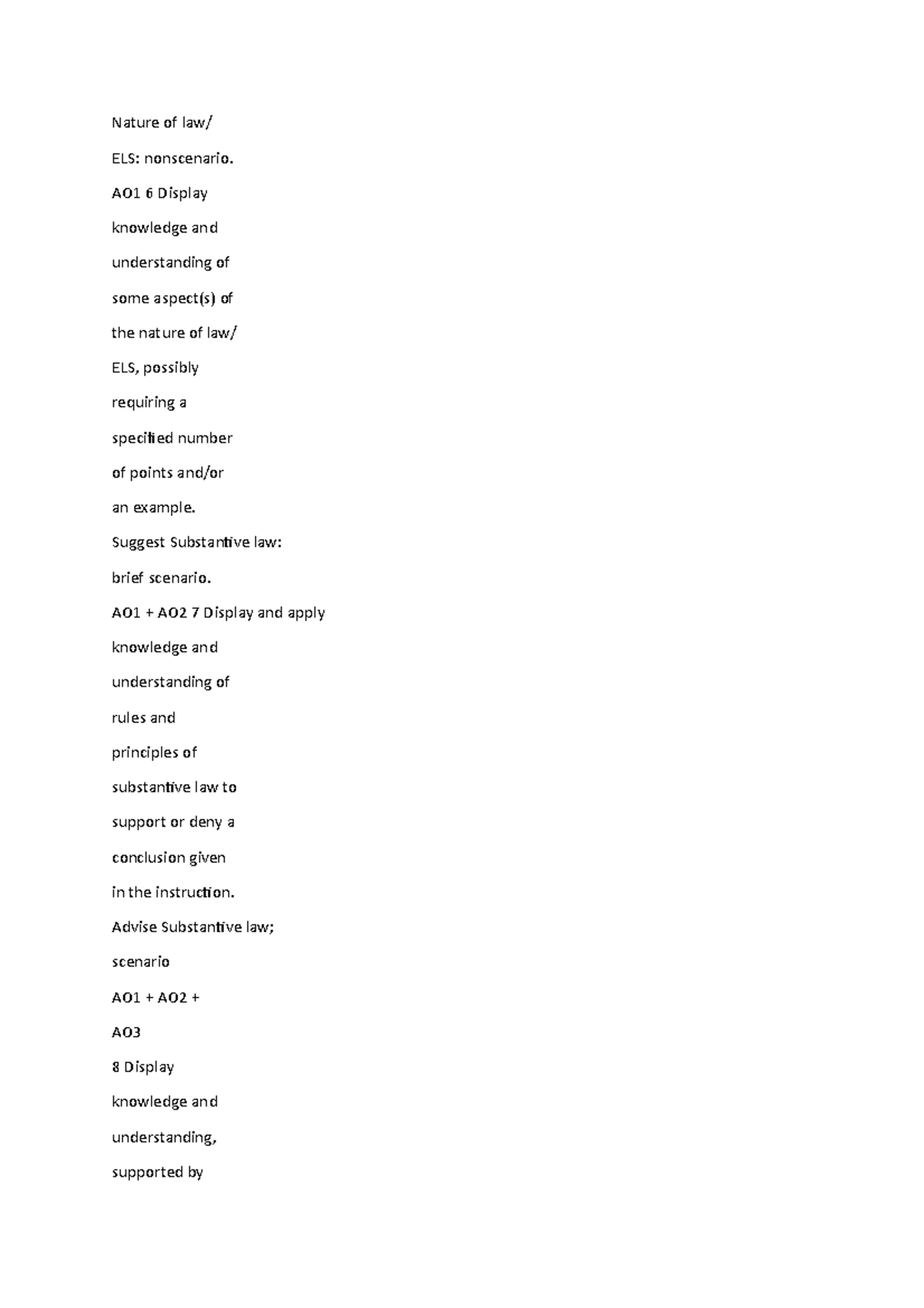**Descriptive Caption:**

The image displays a vertically aligned list of text on a white background, organized into short sentences consisting mostly of two words each. From top to bottom, the text reads:

1. Nature of law
2. ELS
3. AO1 6 display
4. Knowledge and
5. Understanding of
6. Some aspects of
7. The nature of law
8. ELS possibly
9. Requiring a specified
10. Number of points
11. Enter an example
12. Suggest substantive law
13. Brief scenario AO1 plus AO2 7 display
14. Apply
15. Knowledge and understanding
16. Rules and principles of
17. Substantive law to support or deny a conclusion
18. Given on the instruction
19. Advice substantive law scenario AO1 plus AO2
20. AO3
21. B display
22. Knowledge and understanding
23. Supported by

The entire content is set against a plain white backdrop, which makes the text stand out starkly, emphasizing its instructional and explanatory nature.